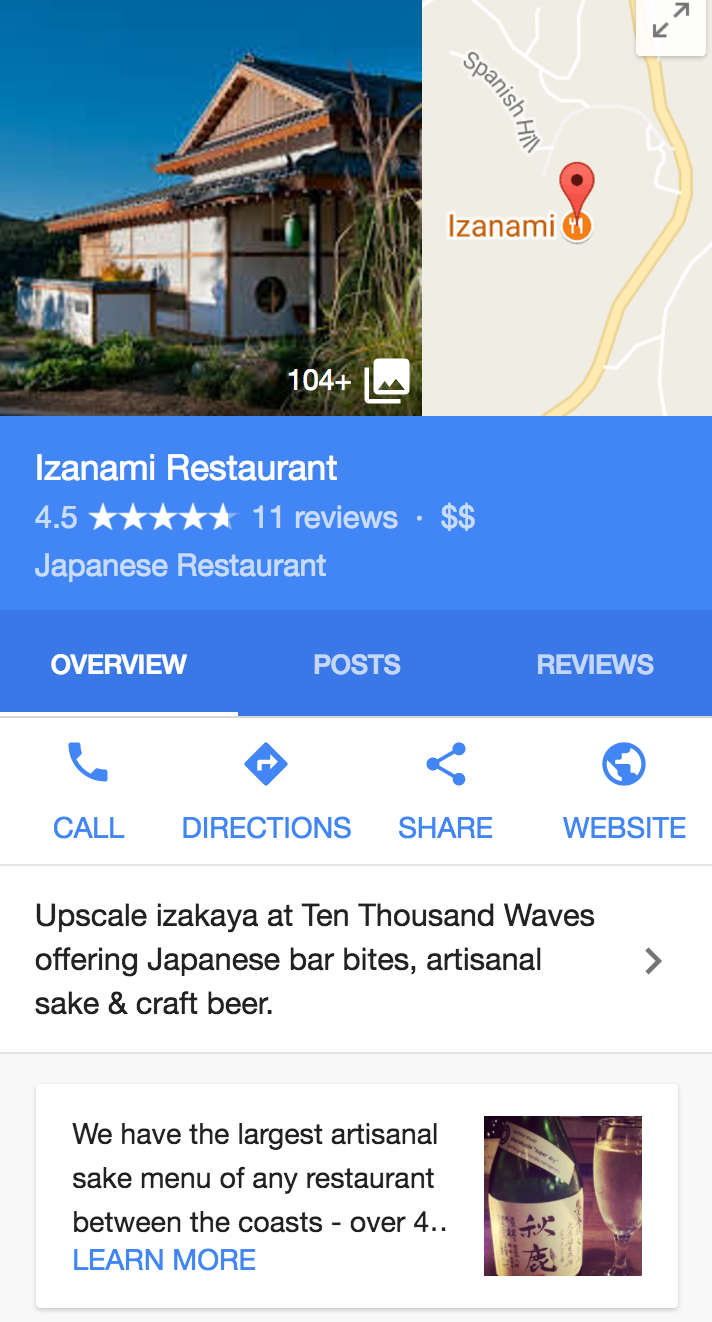This is a detailed, cleaned-up descriptive caption for the image:

"An image of a restaurant overview displayed on a mobile interface. The background features a blue gradient transitioning to a slightly darker blue near the bottom. On the left side, there's a photograph showing the exterior of Izanami, a Japanese restaurant rated 4.5 stars from 11 reviews, designated by two dollar signs ($$). The restaurant has over 104 additional photos available. On the right side, there's a map location. Various tabs—Overview, Posts, and Reviews—are shown with the Overview tab highlighted. Below this section, on a white background with blue text, options to Call, Get Directions, Share, and Visit Website are displayed.

The restaurant is described as "upscale izakaya at 10,000 Waves, offering Japanese bar bites, artisanal sake, and crafted beers," with an arrow directing users to more information. There's also a promotional rectangle stating, "We have the largest artisanal sake menu of any restaurant between the coasts. Over..." followed by a truncated invitation to "Learn more." Adjacent to this text is a photograph of a bottle of sake and a glass of sake, presented in a wine glass, adding to the aesthetic appeal of the beverage offering. The composed layout and vibrant colors create a visually engaging and informative presentation."